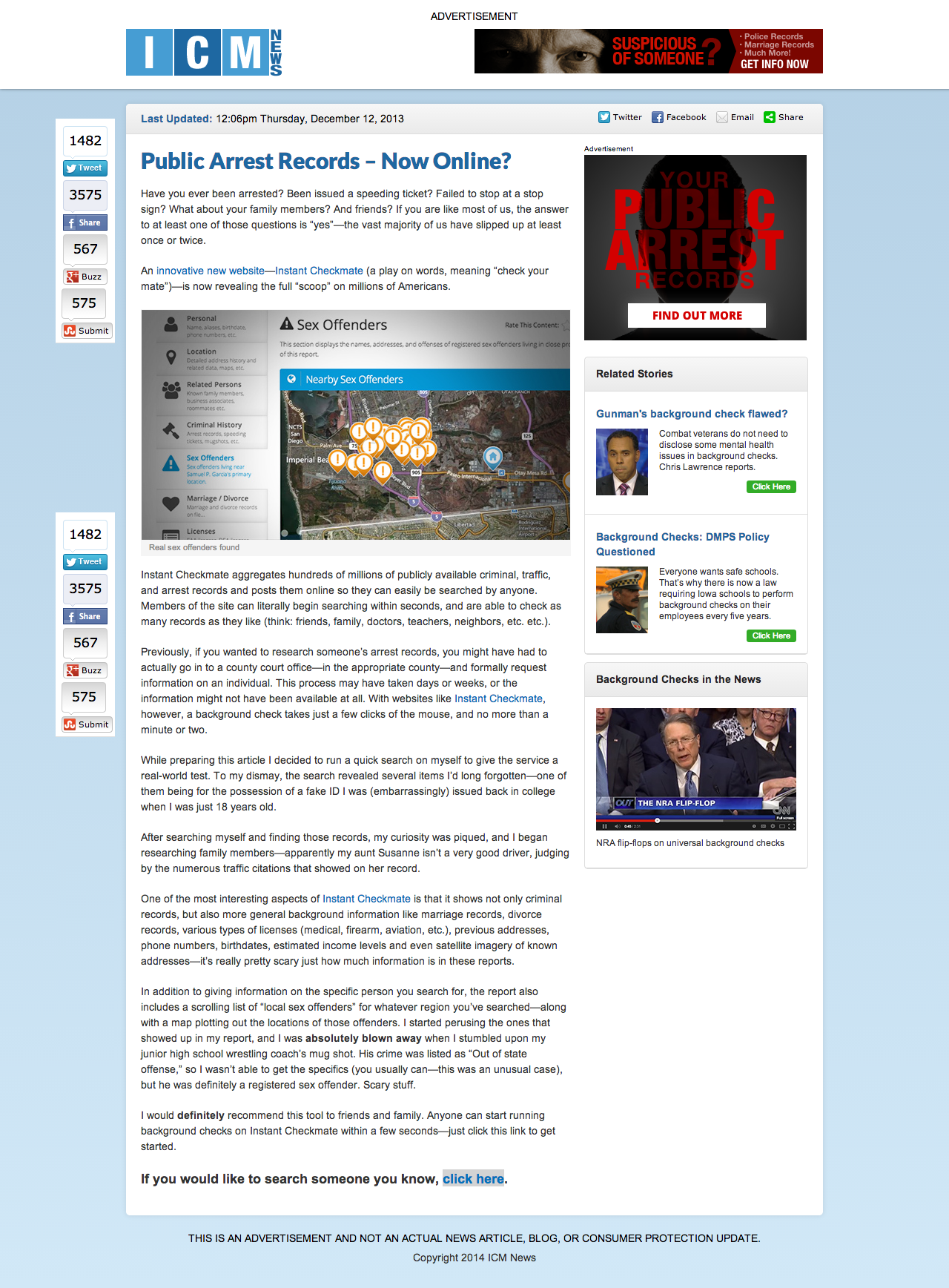**Detailed Caption:**

This image is a screenshot of the website ICM News, which prominently features an advertisement for Instant Checkmate, a background check service. At the top of the page, the banner "ICM News" is displayed, accompanied by an image of a man's frowning face covering the upper portion of the screen. To the right of the banner, a call-to-action reads, "Suspicious of someone? Police records, marriage records, much more, get info now."

The ad announces that the content was last updated at 12:06 p.m. on Thursday, December 12, 2013. It highlights, "Public arrest records now online," and begins with a series of questions like "Have you ever been arrested, been issued a speeding ticket, failed to stop at a stop sign? What about your family members and friends?" This teaser seeks to engage users by pointing out that most people have some sort of record.

The article within the ad explains how Instant Checkmate aggregates hundreds of millions of publicly available records, including criminal, traffic, and arrest records, making them easily searchable online. It emphasizes that members can begin their searches within seconds and can check unlimited records for friends, family members, doctors, teachers, neighbors, and more.

Previously, such searches required a formal procedure at county court offices, which was time-consuming and sometimes unfruitful. Instant Checkmate claims to solve this by providing comprehensive reports within minutes, detailing not only criminal records but also general background information such as marriage and divorce records, various licenses, addresses, phone numbers, birth dates, income levels, and satellite imagery of known addresses.

The testimonial portion reveals the author's personal experience using the service, discovering forgotten incidents such as a college-era fake ID citation and uncovering family members' traffic violations. Furthermore, it describes an in-depth look at the reports' features, including scrolling lists and maps of local sex offenders, with an alarming personal revelation about the author's junior high school wrestling coach being a registered sex offender.

The ad concludes with a recommendation for the tool and provides clickable links for users to start their own background checks. 

To the right side of the page, there are additional related headlines about background checks, such as "Gunman's background check flawed," "Combat veterans do not need to disclose some mental health issues in background checks," and “NRA flip-flops on universal background checks,” among others.

At the bottom of the screenshot, a disclaimer states, "This is an advertisement and not an actual news article, blog, or consumer protection update," followed by the copyright © 2014 ICM News.